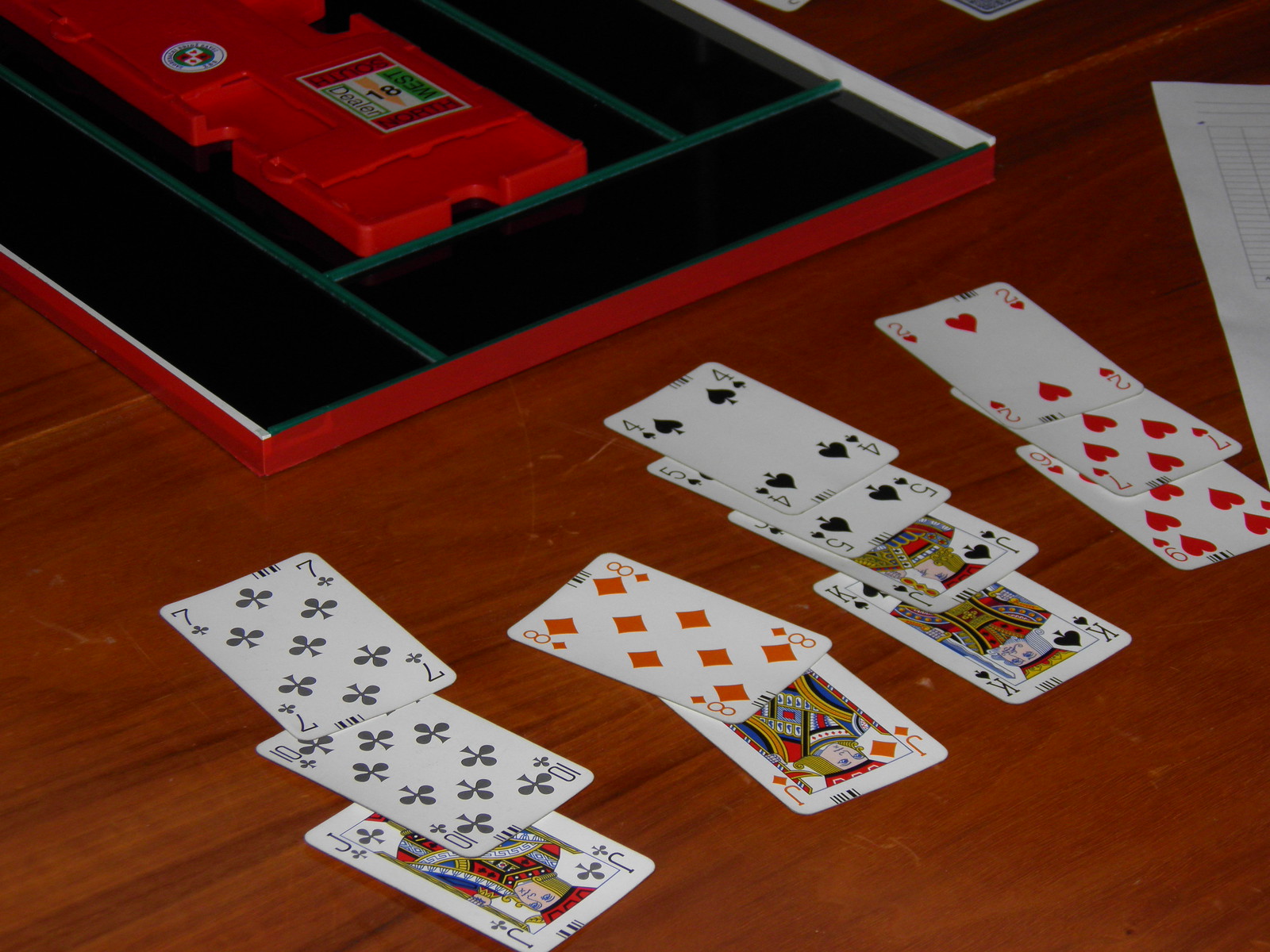This detailed photograph captures a wooden tabletop with a rich reddish-brown hue and dark brown grain patterns. In the upper left corner, there is a unique item resembling a large picture frame with a metal grate embedded in it. Sitting atop this frame is an irregularly shaped red plastic object featuring various openings and unusual forms, as well as a label that reads "18" among some obscured text.

Centered on the tabletop is a game of solitaire in progress. The arrangement of playing cards is meticulously detailed, starting with a row on the left side consisting of the seven of spades, the ten of spades underneath, and the jack of spades beneath that. Adjacent to this row is the eight of diamonds placed on top of the jack of diamonds. Continuing towards the right, there is another row beginning with the four of spades, followed by the five of spades, the jack of spades, and the king of spades.

The next row then starts with the two of hearts, followed by the seven of hearts, and concluding with the nine of hearts. The image captures the intricacies of the playing cards and the layered texture of the wooden tabletop, forming a vivid and evocative scene.